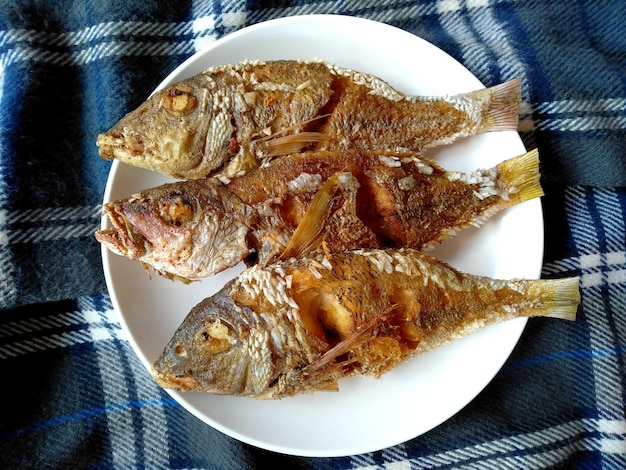The image depicts a close-up of a white round plate resting on a wavy, blue plaid tablecloth. Atop the plate are three small, whole fish that have been prepared in a deep fryer, exhibiting a golden crisp exterior. The fish are a mix of tan, brown, orangey, and yellow hues, and they lie aligned with their heads pointing to the left. Despite the different degrees of frying, all three still retain their scales and tails, though two lack eyes and one has a naturally gray head. The setting appears to be indoors, potentially for a food presentation or a cookbook photo, given the composition and details. The plate and fish are surrounded by contrasting colors of brown and blue, adding vibrancy to the overall arrangement. Some white residue is visible on the fish, the nature of which is unclear.